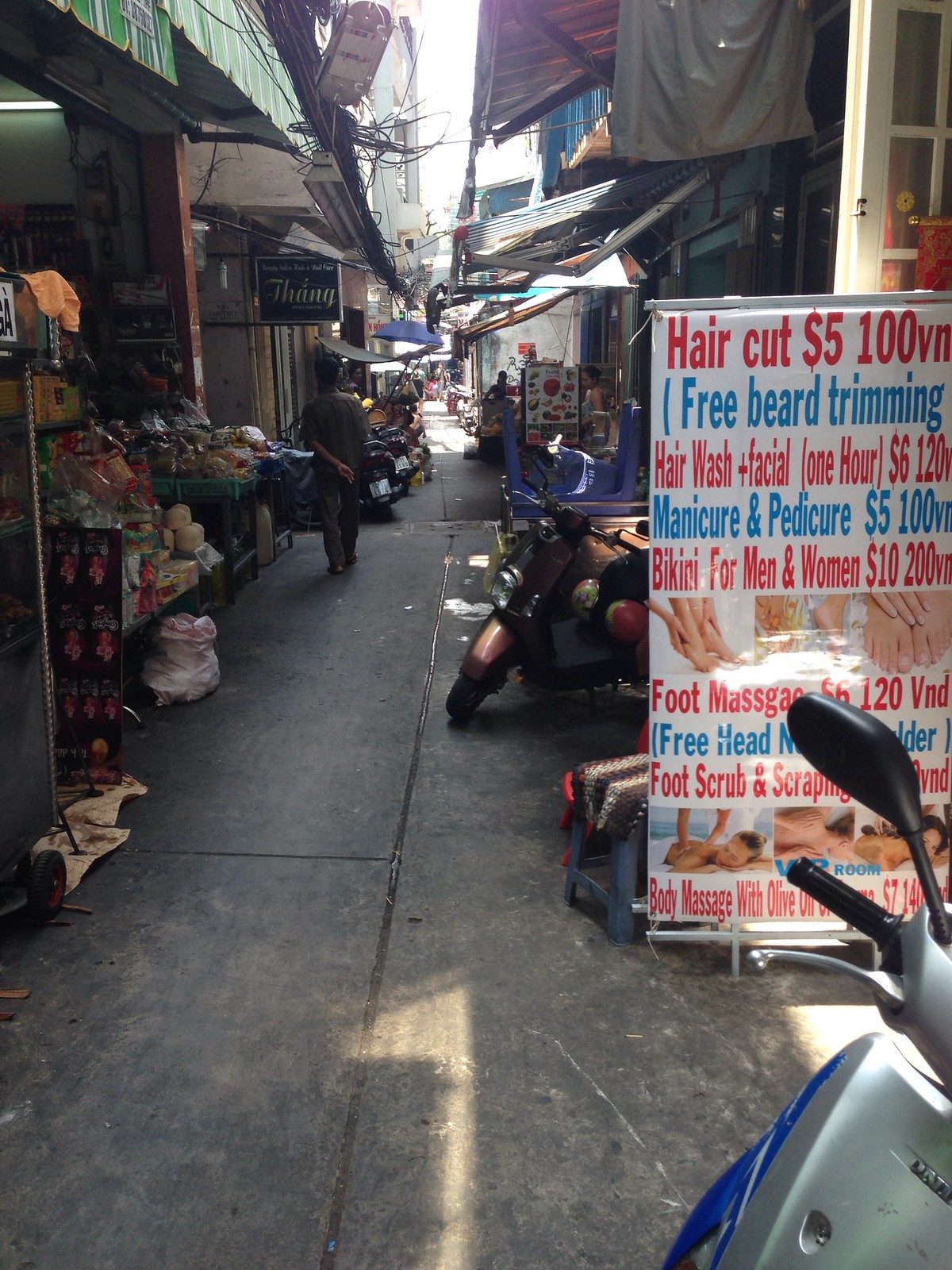The image depicts a vibrant and bustling outdoor marketplace, reminiscent of a narrow alleyway, likely situated in a developing country. The scene unfolds in broad daylight, revealing a gray stone walkway that runs up the center of the image, flanked by various storefronts and street vendors offering an array of services and goods. Prominently centered on the right side of the image is a colorful sign in red, white, and blue text, advertising a variety of affordable personal care services: "haircut $5, free beard trimming, hair wash, facial, manicure and pedicure, bikini for men and women, foot massage, foot scrub and scraping." The marketplace appears void of people at the moment, with numerous parked motorbikes and scooters lined along the sides of the walkway, suggesting it could be the end of the day or early before business hours. Overhead, a tangle of wires stretches across the narrow street, adding to the sense of an authentic, lively market scene. The color palette of the image includes shades of gray, blue, red, white, light blue, orange, yellow, black, and green, contributing to the vibrant atmosphere of this open-air market.